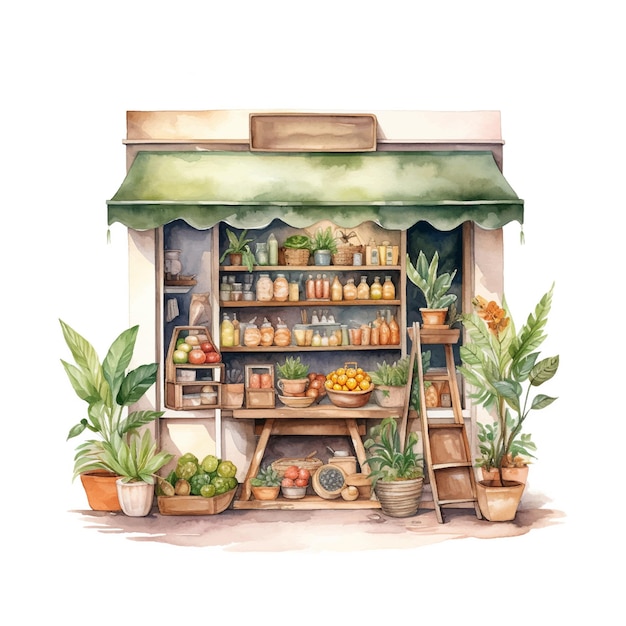This detailed watercolor painting depicts an outdoor market stand, set against a white background. The stand features a deep green awning extending over the shelves, which are filled with various bottles and jars, predominantly in yellowish-orange hues, along with small potted plants. Above the awning is a blank wooden sign attached to a light yellow or off-white facade. The market stall includes a central section with four neatly stacked shelves and two side sections with one or two shelves each. Loose arrangements of fruits, vegetables, and terracotta pots of greenery are placed on these shelves, with the central setup bolstered by a four-legged wooden table holding a bowl of lime-like fruits and various potted plants, potentially herbs. The ground in front of the stand is dotted with verdant floor plants in terracotta and light white stone clay pots, with some featuring bright red flowers, possibly hibiscus or bird of paradise. To the right, a wooden step stool or ladder holds additional pots of greenery. The lower foreground area of the painting suggests a sidewalk, completing this charming, intricately detailed scene of an inviting market stand.